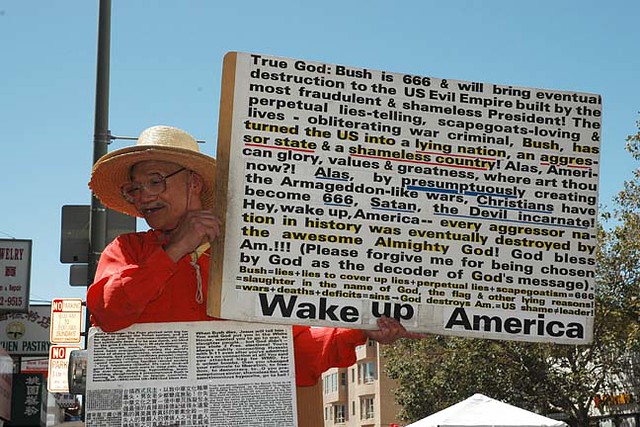In the image, a man in a straw hat is wearing a long-sleeve red shirt while holding up a large, thick sign. The man, positioned to the left of the frame, is looking down and to his left, grasping the sign with his left arm underneath the middle and his right hand near the lower end. The sign features approximately 16 lines of black print, with select phrases underlined in red or blue, and three lines of smaller print beneath. The prominent black text at the bottom reads, "Wake up America." The detailed message on the sign includes statements like "True God, Bush is 666," and accuses former President Bush of turning the U.S. into a nation of lies and aggression, calling him a war criminal. Further text expresses that Christians have become "666, Satan, the devil incarnate" due to Armageddon-like wars. The background includes buildings, trees, a large street sign pole, and billboards, giving context to what appears to be a protest scene.